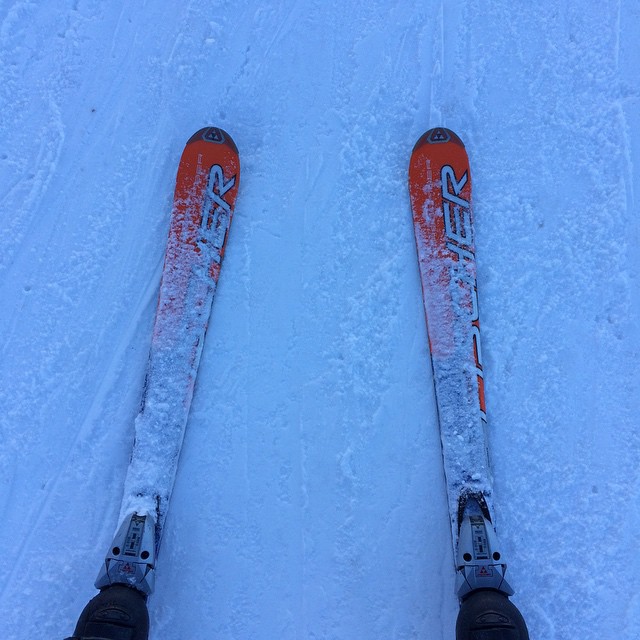In this image, we see a person's partially visible feet in black snowboard boots securely strapped into a pair of skis. The scene is set on a snowy surface with noticeable striations, suggesting a frequently skied or groomed area. The skis, predominantly vibrant orange with some parts obscured by snow, feature a triangular logo formed by three smaller triangles near their tips, which appear more brown. Underneath the snow on the skis, there's partially visible text that might spell out "Fischer" in white lettering, though obscured by accumulated snow. The day appears dark and cloudy with minimal sunlight, contributing to the overall dim and blue-tinted appearance of the snowy background.